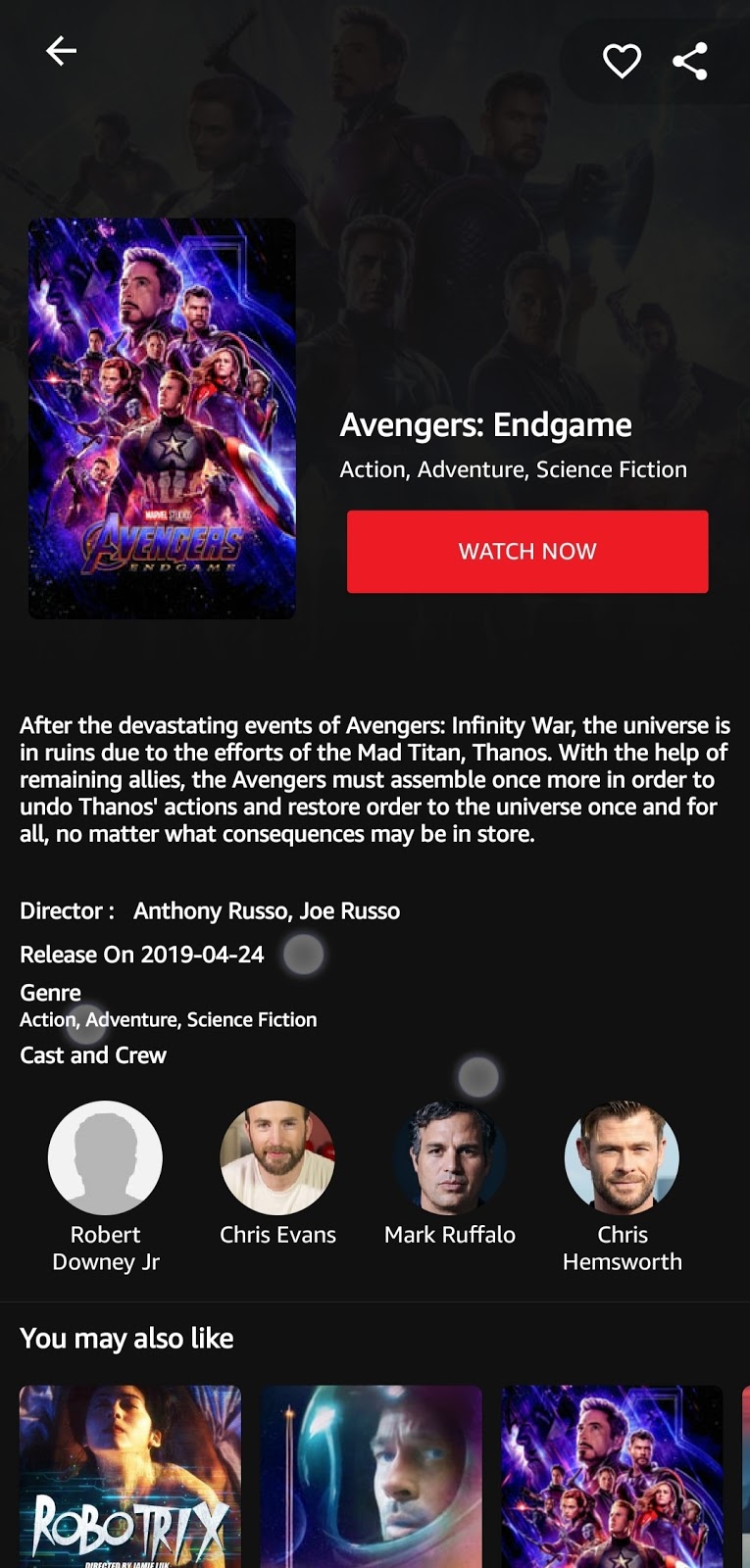The screenshot features a webpage reminiscent of Netflix, showcasing an advertisement for the movie "Avengers: Endgame." Dominating the page is a smaller version of the iconic movie poster for "Avengers: Endgame," positioned prominently. Adjacent to it, the title "Avengers: Endgame" is displayed in a bold white font. Beneath the title, the genres "Action, Adventure, Science Fiction" are listed, hinting at the film's dynamic content.

Further down, a prominent red rectangle with the directive "Watch Now" in white font beckons viewers to either purchase access or, if already subscribed, start streaming the movie immediately. Below this call-to-action, there is a brief synopsis of the movie in white text, providing a quick glimpse into the film's storyline.

The webpage also includes detailed information about the film, such as the director's name, release date, genre, and notable cast and crew members. Accompanying this information is a series of circular thumbnail images featuring members of the cast, offering a visual introduction to the stars of the film.

At the very bottom of the screen, a "You May Also Like" section displays a horizontal bar of similar movies, suggesting additional content that fans of "Avengers: Endgame" might enjoy.